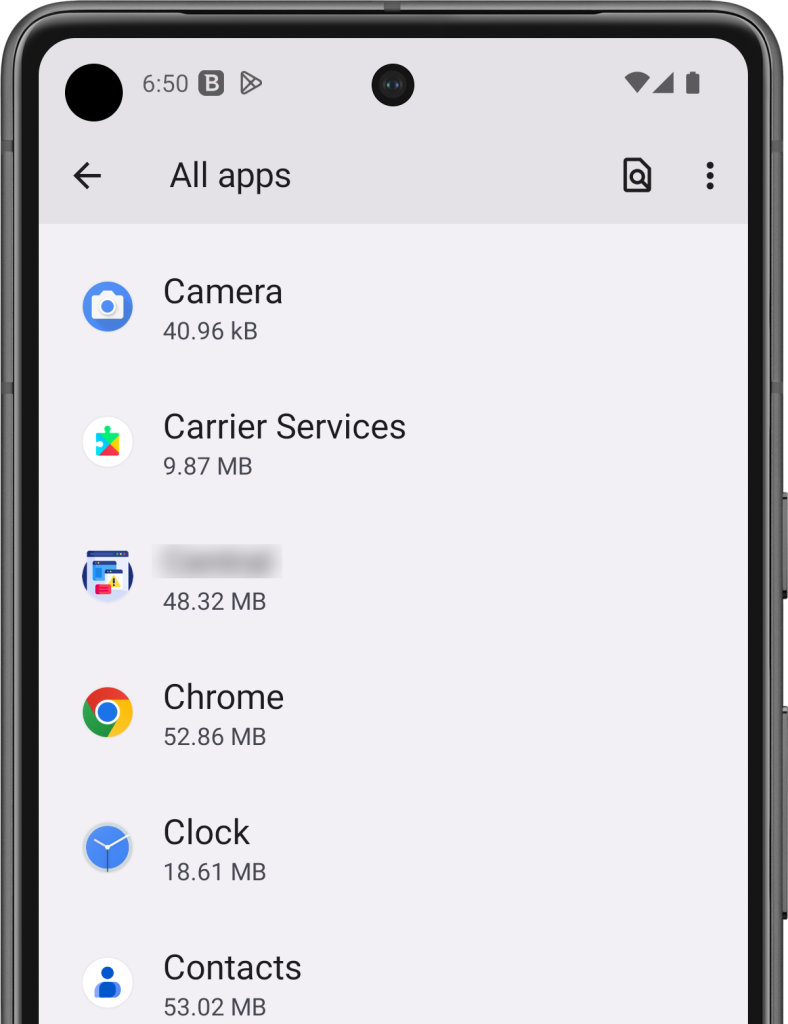This is a detailed screenshot of an Android phone's Apps Drawer, accessed through the All Apps section in the settings menu. The screenshot showcases a series of apps, notably displaying the Camera app at the top followed by the Carrier Services app. Beneath these is an app with its name blurred out, sized at 48.32 MB, and featuring an unrecognizable logo. Further down the list, visible apps include Chrome, Clock, and Contacts. The screenshot was captured at 6:50, as indicated by the time displayed on the screen. Additionally, the notification bar at the top shows icons for Blogger and Google Play Store, suggesting recent notifications from these apps. The purpose behind the blurring of one app's name remains unclear, possibly for privacy reasons despite it being merely an installed application.